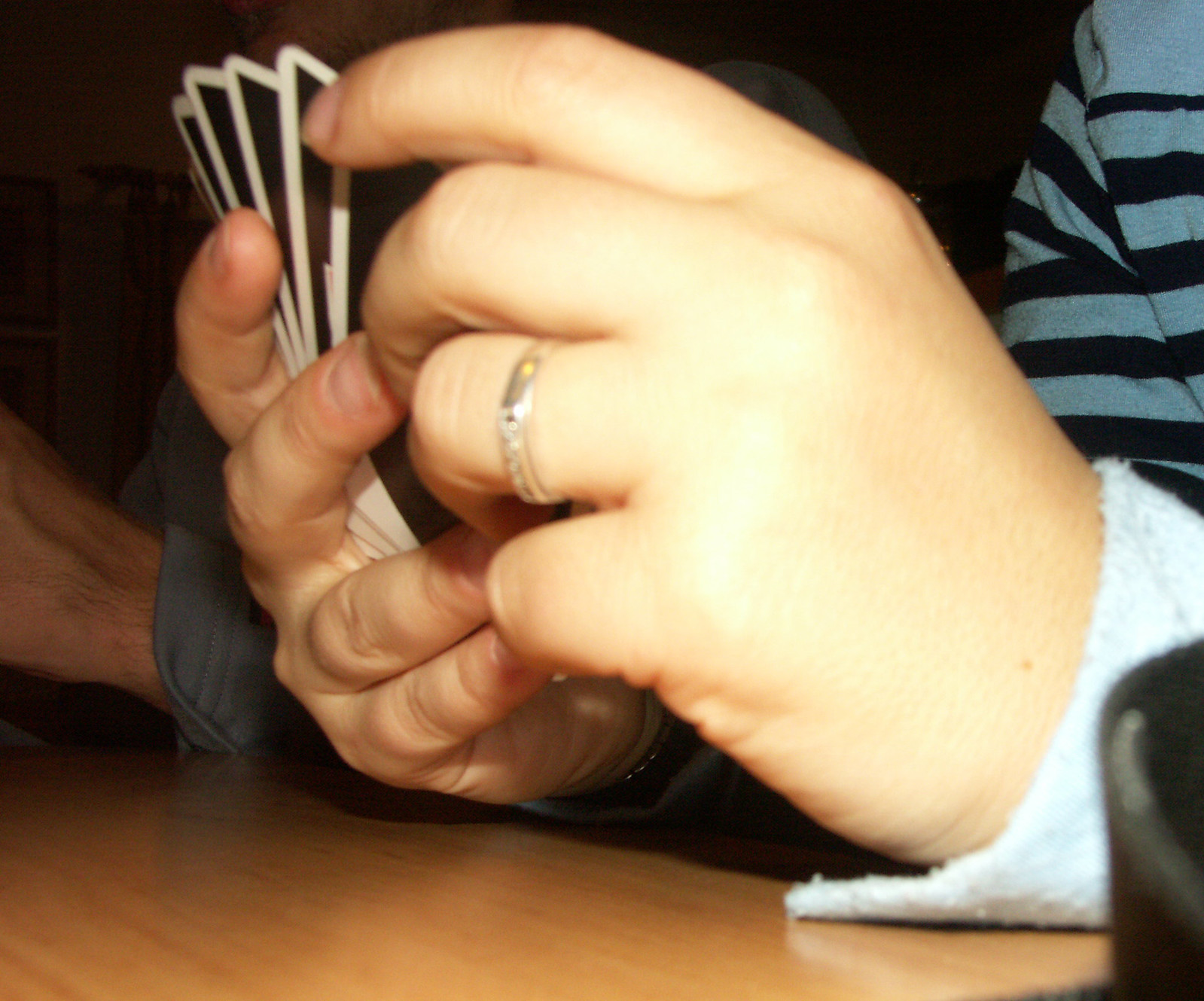In this close-up image, we see a pair of chubby, thick hands with a wedding band on the ring finger of the left hand, suggesting they might belong to a woman despite their masculine appearance. The hands are positioned towards the left side of the image, indicative of the person being mostly in profile facing that direction. They are holding a set of Uno cards, distinctively black with white borders. The individual is wearing a light blue long-sleeved shirt adorned with navy blue stripes. Their hands are resting on a light brown wooden table. In the dimly lit background to the left, another person is visible, also clad in a long-sleeve blue shirt, with some hair on their hands and wrists, suggesting a man. The overall scene has a cozy, intimate feel, with the engaged players deeply absorbed in their game.